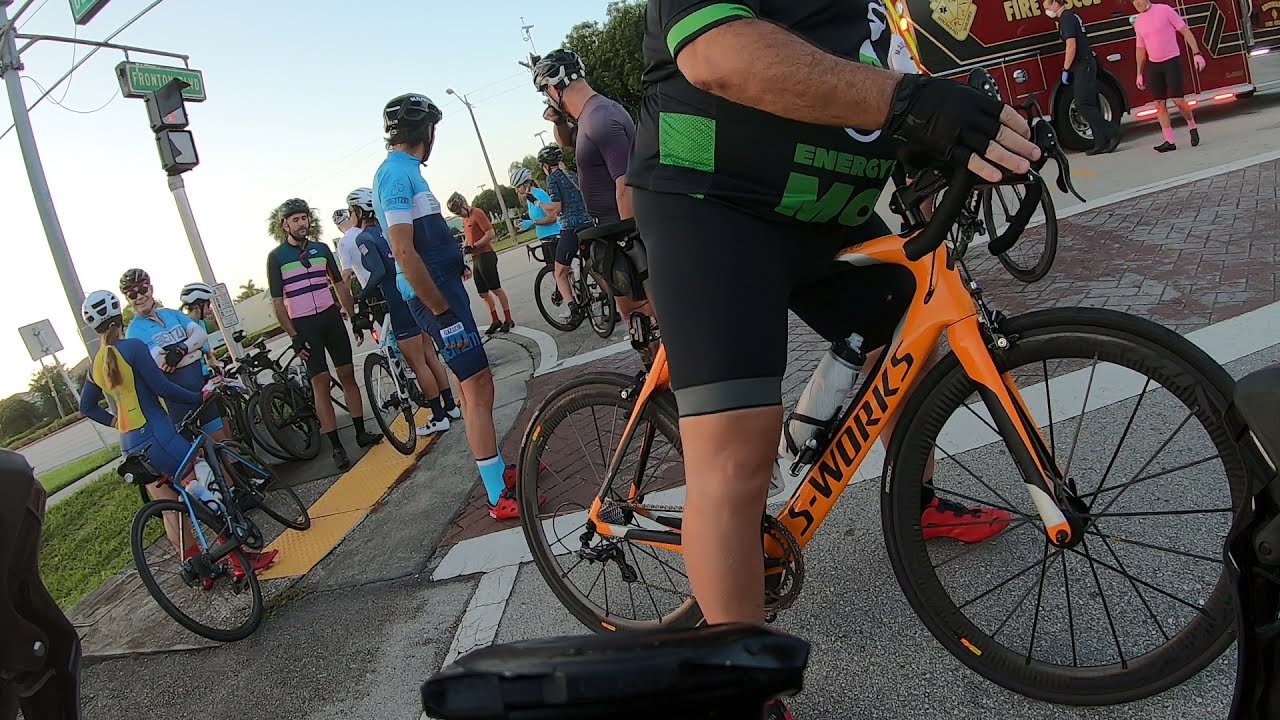In this image, we see a bustling outdoor scene set on an asphalt road enhanced with patches of brick at the bottom. Dominating the scene are several bicyclists, all wearing helmets and sunglasses, suggesting a focus on safety. They appear to be in a group, possibly conversing or assessing a recent event. The most prominent individual is seated on a striking bright orange bike labeled "S-Works" on the bottom frame, which also features sleek black rims. This gentleman is outfitted in black biking gloves with cut-out fingers and black shorts with a gray band above the knee. Surrounding him are roughly 10 to 12 other cyclists, some engaged in conversation.

A fire truck is noticeable in the top right corner of the image, raising questions about whether it’s parked there due to an incident or simply adjacent to a nearby fire station. Street signs are scattered throughout, but the image isn’t centered on any specific object, giving a more holistic view of the event. The color palette is diverse, featuring shades of black, orange, green, tan, light blue, dark blue, pink, and yellow. Overall, the setting appears to be outdoors in broad daylight, capturing a moment of shared focus and interaction among the cyclists.